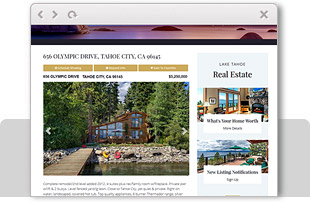This image is a small screenshot of a web browser displaying a website. Due to the reduced size, the text is difficult to read. The browser interface includes a gray bar at the top with standard navigation icons: a less-than arrow and greater-than arrow, suggesting back and forward buttons, accompanied by a circular arrow likely representing the refresh function. On the far right of this bar, there's a dark gray 'X' icon indicating the close window feature.

Beneath the browser bar, a vivid banner stretches across the page, displaying a colorful landscape that appears to be an ocean scene in hues of purple and pink. In the center of the page, there's an undecipherable image with the text "Olympic Drive, Tahoe City" above another indistinct image, perhaps of a cabin. 

On the right side of the page is a section titled "Lake Tahoe Real Estate," accompanied by two images, presumably depicting properties available in the Lake Tahoe area. Due to the image's small size, the finer details and additional textual information are not legible, but the screenshot provides a glimpse into a real estate website focused on properties in the Lake Tahoe region.